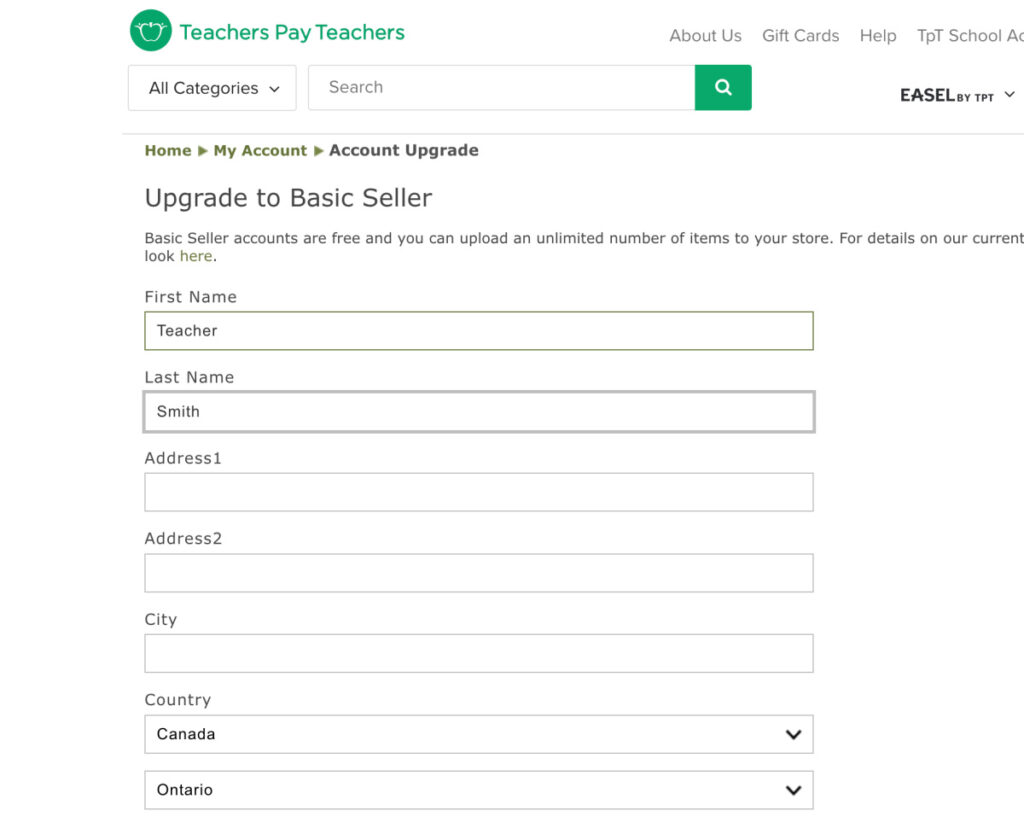In this image, there is a screenshot from a website. At the top left corner, there is a circular logo featuring a white drawing on a green background. Next to the logo, the words "Teachers Pay Teachers" are written in green font. On the same horizontal line, but on the right side, there are multiple buttons labeled "About Us," "Gift Card," "Help," and "TPT School AC," with the text in light grey.

Below this line, on the left, there is a drop-down menu labeled "All Categories," indicating that the user can select different categories, but currently, "All Categories" is selected. Adjacent to this is a search bar with the word "Search" inside it, alongside a white search icon on a green background. 

Further down, breadcrumb navigation shows the path "Home / My Account / My Account Upgrade." Beneath this, there is a prompt to "Upgrade to Basic Seller," instructing users to fill in their details. Most of the text in this section is written in grey ink.